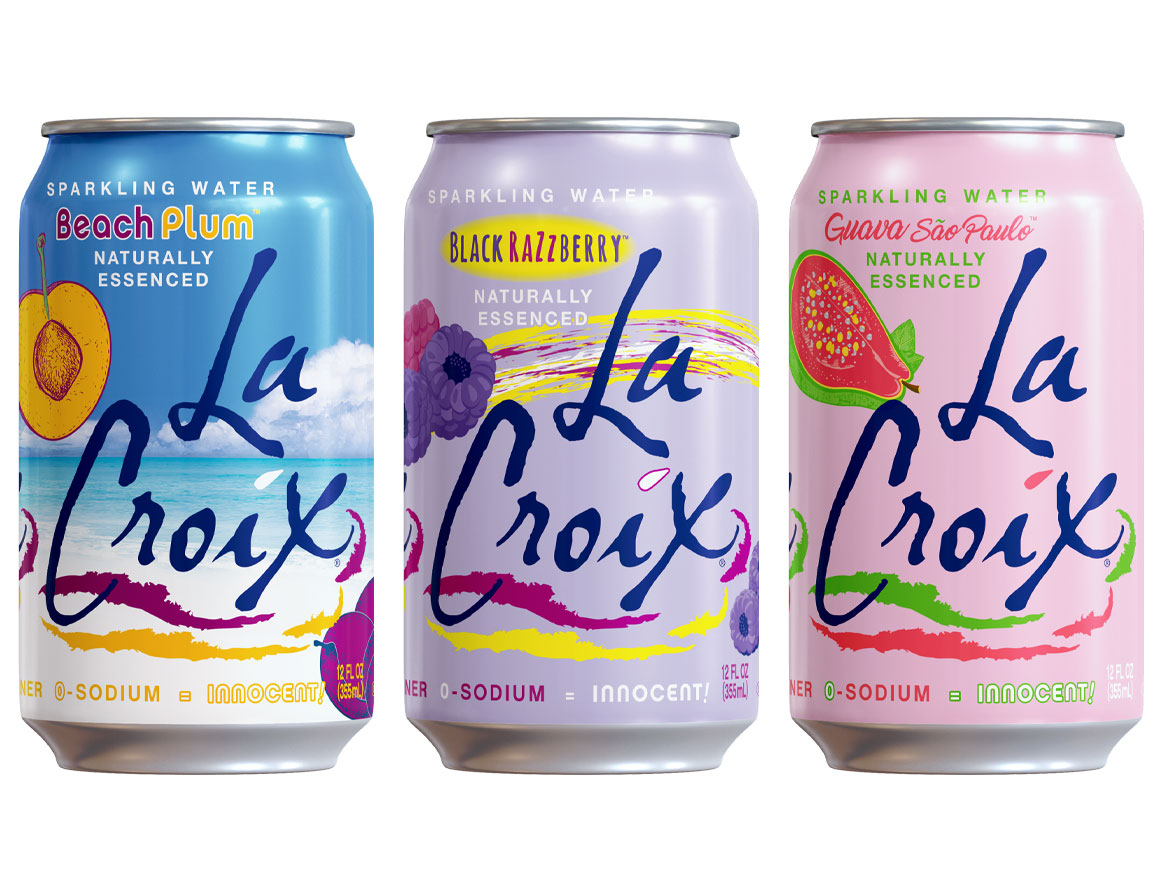This photograph captures three La Croix sparkling water cans, each featuring distinctive and colorful designs. The cans resemble traditional aluminum soda cans but feature vibrant and beach-inspired imagery. Starting from the left, the first can showcases a blue sky with white clouds, a beach setting, and an illustration of a plum, representing the Beach Plum flavor. The can reads, "sparkling water beach plum naturally essenced," and highlights the brand’s signature message, "zero sodium equals innocent."

In the center, the second can is adorned with light purple hues and images of deep purple raspberries, reflecting its Black Raspberry flavor. It also includes the text, "sparkling water black raspberry naturally essenced," and features the same La Croix logo in bold, handwritten-style blue letters.

The final can on the right is designed with a light pink background accented by green highlights, depicting a guava. This can promotes the Guava Sao Paulo flavor and carries the familiar branding, "sparkling water guava Sawa Palo naturally essenced," along with the consistent tagline, "zero sodium equals innocent." Each can contains 12 fluid ounces of naturally essenced sparkling water, showcasing La Croix’s distinctive branding across varied yet cohesive visual themes.